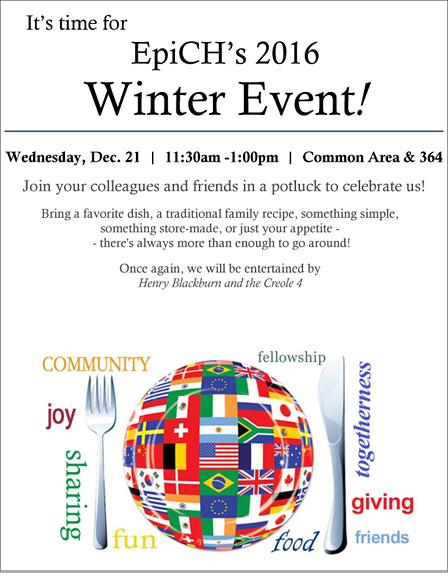This advertisement flyer for EPIC's 2016 Winter Event is set against a white background and prominently features black and gray text. It invites colleagues and friends to celebrate in a potluck on Wednesday, December 21st, from 11:30 a.m. to 1 p.m. in the Common Area at room 364. The text encourages participants to bring a favorite dish, whether it's a traditional family recipe, something simple, store-made, or just come with an appetite, assuring that there will be plenty of food to go around. Entertainment for the event will be provided by Henry Blackburn and the Creole Four. The flyer also includes a colorful image of a dinner plate adorned with flags from around the world, symbolizing global community and fellowship. A silver knife and fork flank the plate, and the surrounding text highlights values such as community, fellowship, togetherness, giving, friends, food, fun, joy, and sharing. The colors around the text range from green to blue to red to yellow, adding a vibrant and inviting touch to the overall design.